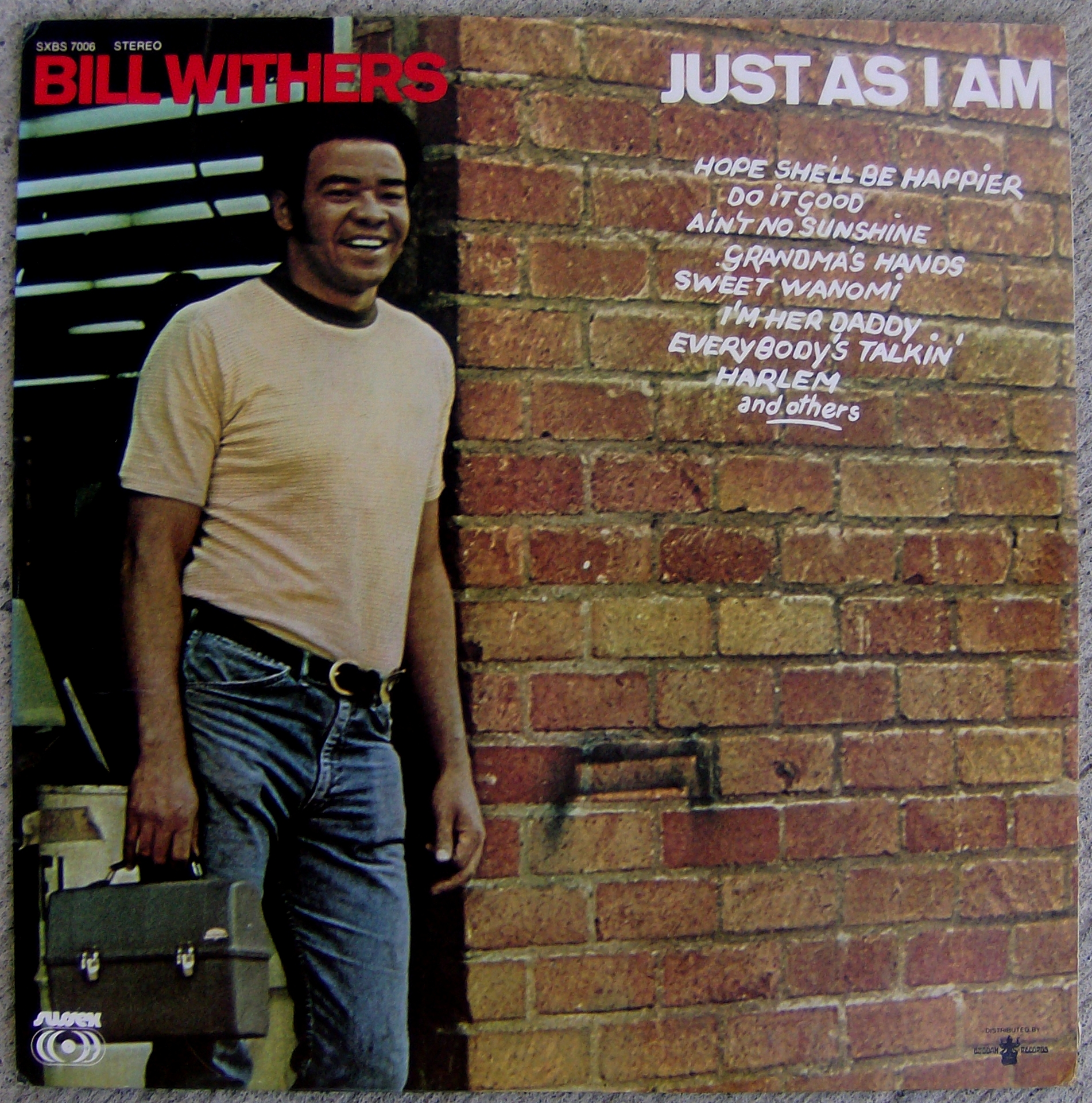This photograph depicts the album cover of Bill Withers' "Just As I Am." The cover shows Bill Withers emerging from a brick building, likely a warehouse, emphasizing his working-class image. He stands on the left side of the cover, leaning against the brick wall with a broad smile on his face. Bill is dressed in a yellow or beige 1970s-style t-shirt, jeans with a visible wallet in one of the front pockets, a black belt with a gold buckle, and holding a gray lunch pail with silver buckles in his right hand. He sports a slight afro with small mutton chops. The left upper corner features the album identification number SXBS7006 and the word "STEREO" above "Bill Withers" written in bold red letters. On the upper right corner, the album title "Just As I Am" appears in white text, followed by a list of some of the songs such as "Ain't No Sunshine," "Grandma's Hands," "Hope She'll Be Happier," "Do It Good," "Sweet Wanomi," "I'm Her Daddy," "Everybody's Talking," and "Harlem." The background includes nondescript barrels and fluorescent lighting, adding to the industrial ambiance. The entire album cover is set against what appears to be a table or countertop. The lower corners contain identifying marks of the recording studio and publisher, albeit difficult to discern due to the photograph's quality and the album's age.